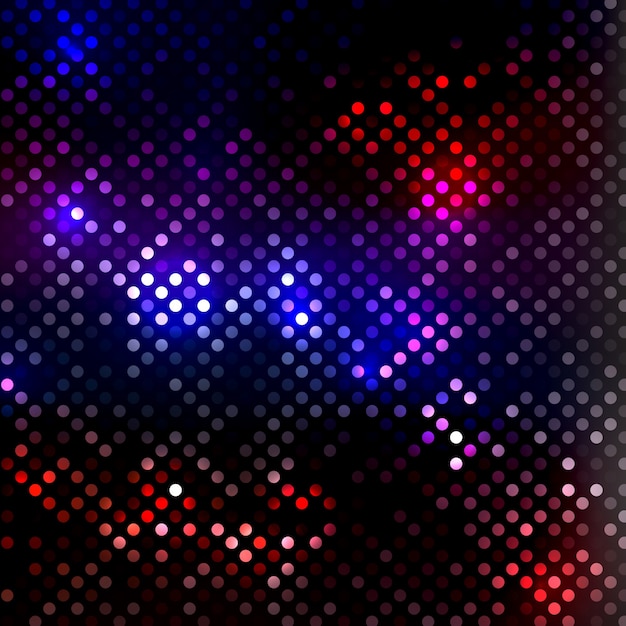The image is an abstract and surreal design featuring a square composition set against a black background. It showcases a series of circles in varying hues and levels of illumination, reminiscent of a glowing Lightbrite toy. These circles are uniformly shaped and sized, emitting light in a spectrum of colors, including blue, red, purple, white, pink, orange, and peach.

In the upper left corner, the circles are predominantly blue, while the upper right corner is marked by red hues. The central area is dominated by blue and purple tones with some white and gray dots interspersed. The bottom third of the image transitions to being mostly red and maroon, accented by occasional white dots, giving the appearance of varying brightness across the design. Some circles appear more illuminated, especially those in the central area, suggesting a dynamic interplay of light within the mosaic-like arrangement. The overall effect is a vibrant and colorful abstract piece with no distinct pattern, blending various shades seamlessly across the canvas.